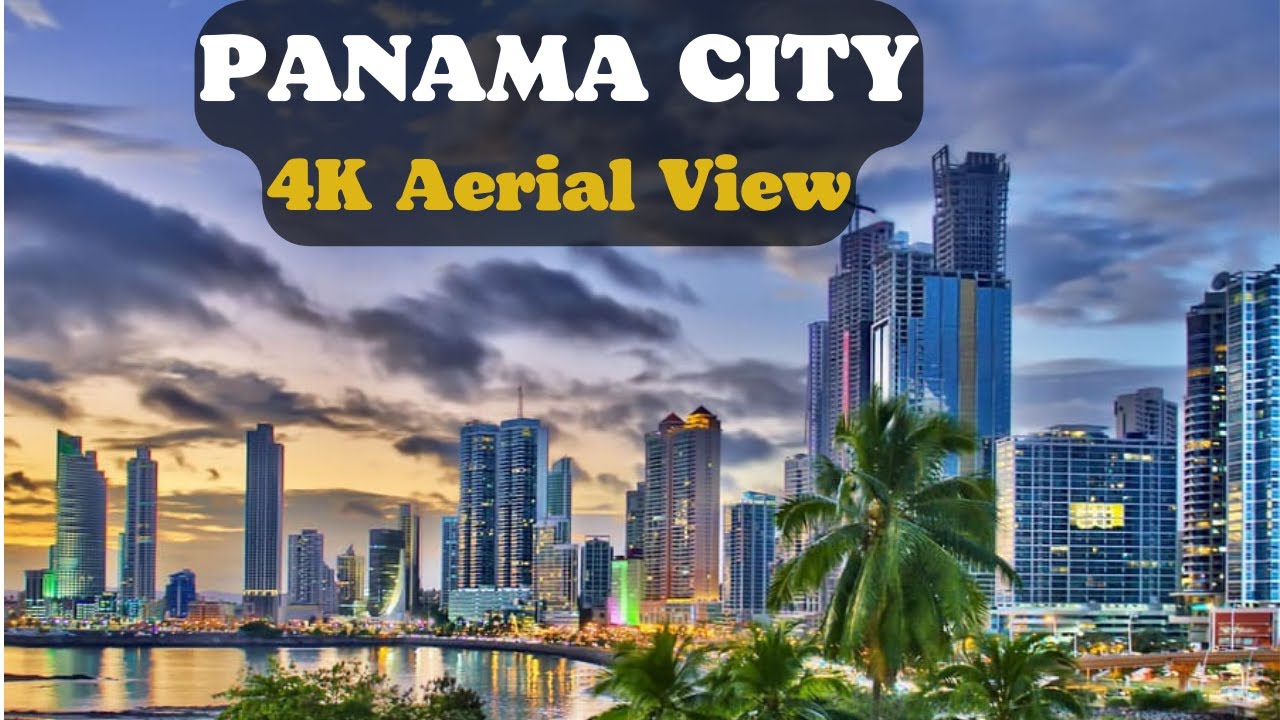The image captures a stunning aerial view of Panama City under a blue sky accented with dark clouds and hints of yellow near the horizon. In the foreground, a prominent black box with white text reads "Panama City" and features "4K Aerial View" in yellow. The background is dominated by illuminated skyscrapers whose lights reflect beautifully on the ocean's surface below. The shoreline is adorned with lush palm trees and several small bushes, adding to the natural beauty of the scene. On the right side of the image, a busy area hints at the city's vibrant activity. Among the buildings, one stands out with a bright, square light in its center, possibly the sun or an intense artificial light, enhancing the picturesque urban landscape. All these elements combine to create a mesmerizing and detailed depiction of Panama City's skyline.